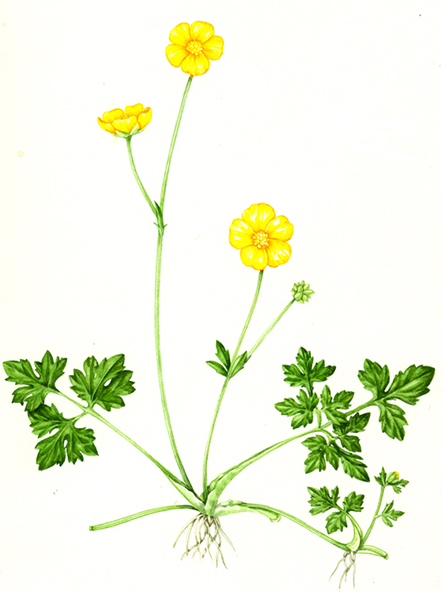The image depicts a detailed hand-drawn picture of a Prickle Seed Buttercup (Ranunculus myrrhachiae). Set against a solid white background, the illustration is vibrant with various shades of green and yellow. The plant features an intricate array of elements: thin green stems rooted at the middle bottom of the image, ornate green leaves spreading out to the left and right of the stems, and three bright yellow flowers that ascend upward. The flowers have shiny yellow petals with darker yellow centers that resemble asters. Notably, a spiky green structure on the rightmost stem hints at the plant's characteristic prickle seeds, which are known to cling to fur and fabric.